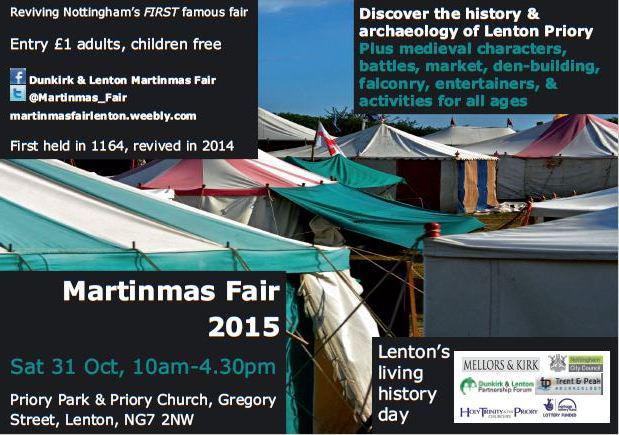This is a vibrant, collage-style flyer advertising the Martinmas Fair 2015, held at Priory Park and Priory Church, Gregory Street, Lenton, NG7 2NW. The centerpiece features a colorful image of green and white, and red and white striped tents under a blue sky. Superimposed on this central image are four insets, each detailing different aspects of the fair. 

In the upper left corner, a black box with white text announces: "Reviving Nottingham’s First Famous Fair, Entry £1 for Adults, Children Free." It also includes social media information: "Facebook: Dunkirk and Lenton Martinmas Fair" and "Twitter: @Martinmas_Fair," followed by the event’s website, "martinmasfairlenton.weebly.com." This inset highlights the fair's historical significance, noting it was "first held in 1164, revived in 2014."

The upper right corner promotes historical and archaeological aspects, stating in white letters: "Discover the History and Archaeology of Lenton Priory," followed by green text listing various attractions: "Medieval Characters, Battles, Market, Den Building, Falconry, Entertainers, and Activities for All Ages."

In the lower left, another black square in white writing marks the event details plainly: "Martinmas Fair 2015," with the date and time highlighted below in green: "Saturday 31 OCT, 10am to 4.30pm."

Lastly, the lower right inset underscores the community aspect, indicating that it takes place during "Lenton’s Living History Day," along with a list of corporate sponsors, also presented in a black box with white text.

The flyer uses a mix of vibrant colors and informational text to effectively promote a day full of historical reenactments, family-friendly activities, and community spirit.